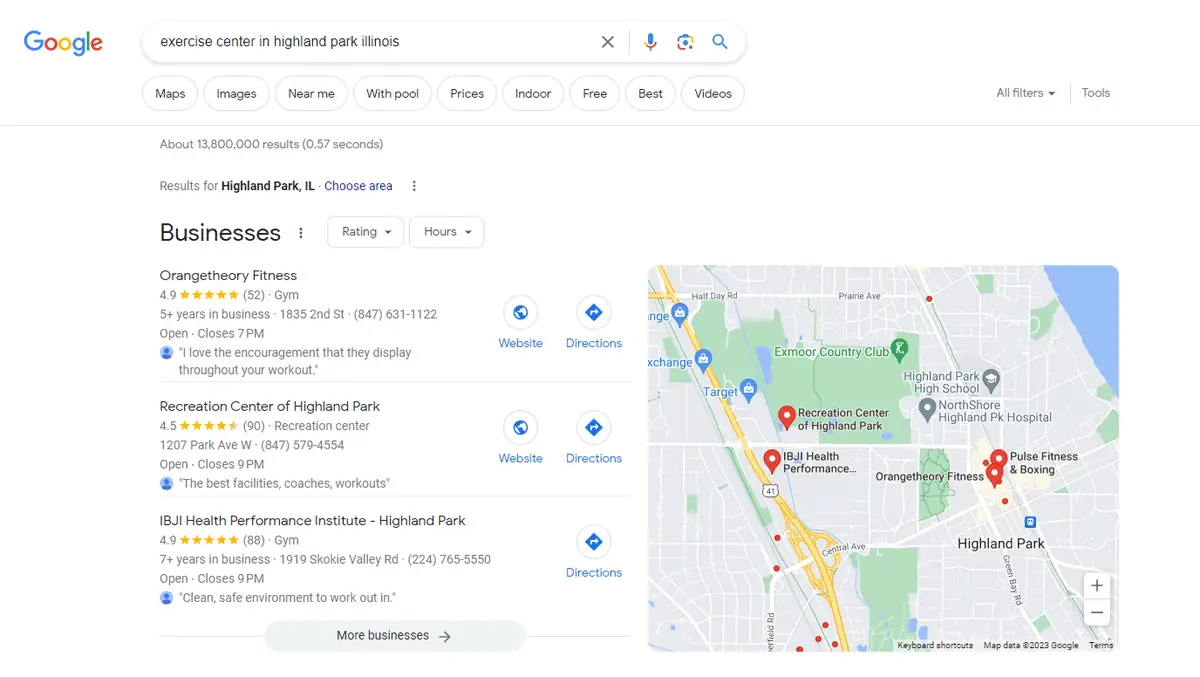This screenshot from Google captures a search results page for "Exercise Center in Highland Park, Illinois." At the top left, the familiar Google logo is displayed in its signature alternating blue, red, yellow, blue, green, and red letters. The search query yields approximately 13,800,000 results in just 0.57 seconds. Various filters such as "Maps," "Images," "Near me," "With pool," "Prices," "Indoor," "Free," "Best," and "Videos" are listed below the search bar.

Detailed information is provided for several local exercise centers:

1. **Orange Theory Fitness**
   - **Rating:** 4.9 stars from 52 ratings
   - **Type:** Gym, more than 5 years in business
   - **Address:** 1835 2nd Street
   - **Phone:** 847-631-1122
   - **Hours:** Open, closes at 7 PM
   - **Review Highlight:** Praised for the encouragement offered throughout workouts
   - **Additional Information:** Website, directions provided

2. **Recreation Center of Highland Park**
   - **Rating:** 4.5 stars from 90 ratings
   - **Type:** Recreation Center
   - **Address:** 1207 Park Avenue West
   - **Phone:** 847-579-4554
   - **Hours:** Open, closes at 9 PM
   - **Review Highlight:** Known for its excellent facilities, coaches, and workouts
   - **Additional Information:** Website, directions provided

3. **IBGI Health Performance Institute**
   - **Rating:** 4.9 stars from 88 ratings
   - **Type:** Gym, more than 7 years in business
   - **Address:** 1919 Skokie Valley Road
   - **Phone:** 224-765-5550
   - **Hours:** Open, closes at 9 PM
   - **Review Highlight:** Clean, safe environment for workouts
   - **Additional Information:** Directions provided

To the right, a map displays the locations of these exercise centers, marked with pins to easily identify their positions within Highland Park, Illinois.